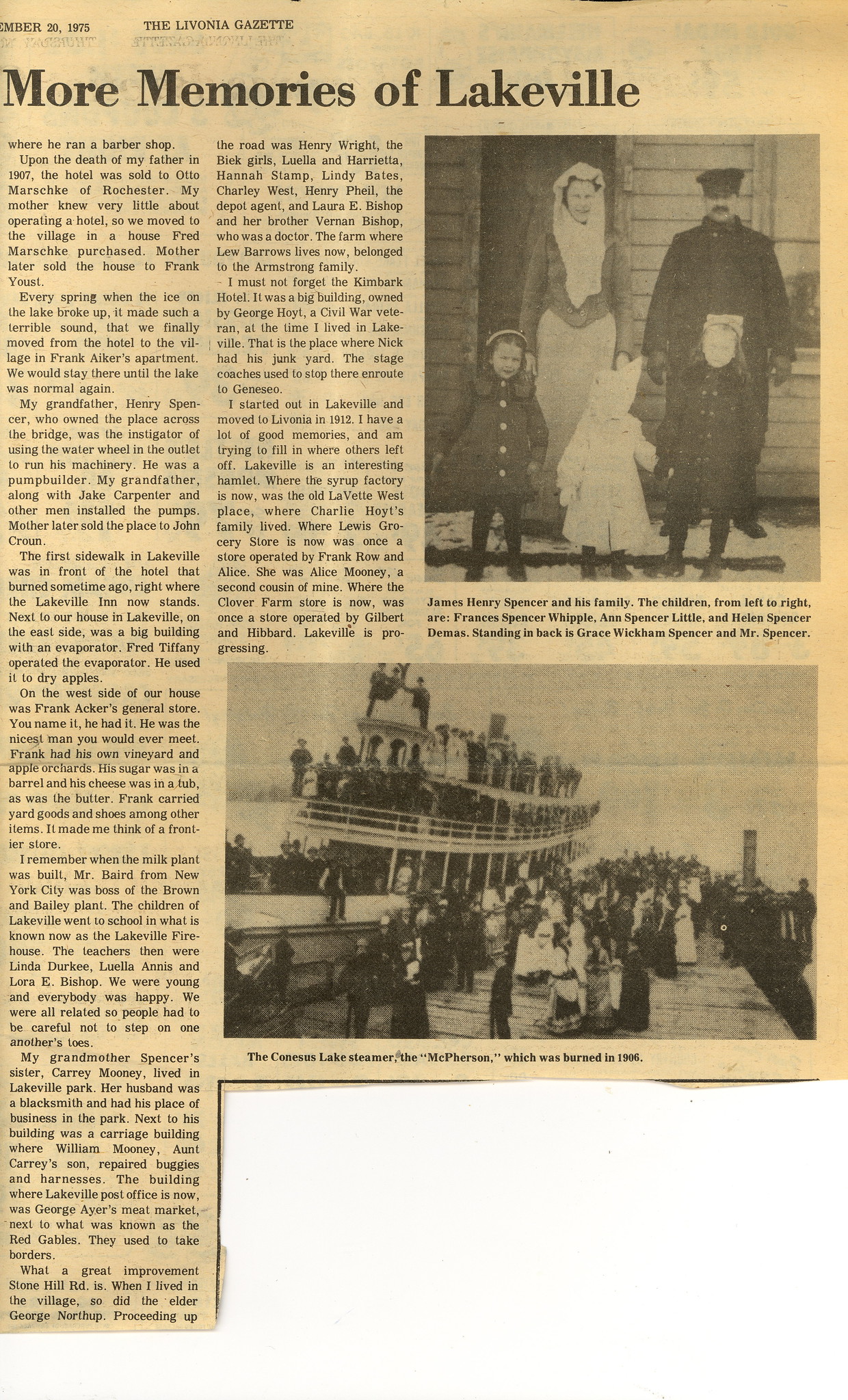This is a photo of an old and weathered newspaper clipping from the Livonia Gazette, titled "More Memories of Lakeville". The paper has yellowed with age, displaying colors like off-white, brown, and gray. The article features two photographs. In the upper right corner, a square photo shows a man and a woman, identified as James Henry Spencer and his family, with three children standing in front of them—all dressed in coats and hats. This image’s setting is unclear whether it was taken indoors or outdoors. Below it, a rectangular photo depicts a bustling dock scene with a boat leaning to its side. The boat, crowded with people, has individuals positioned on its front, back, and sides, while more people wait on the dock. The two-column article includes detailed text: the first column comprises eight paragraphs, and the second has three paragraphs, though the small print is not legible in the photo.